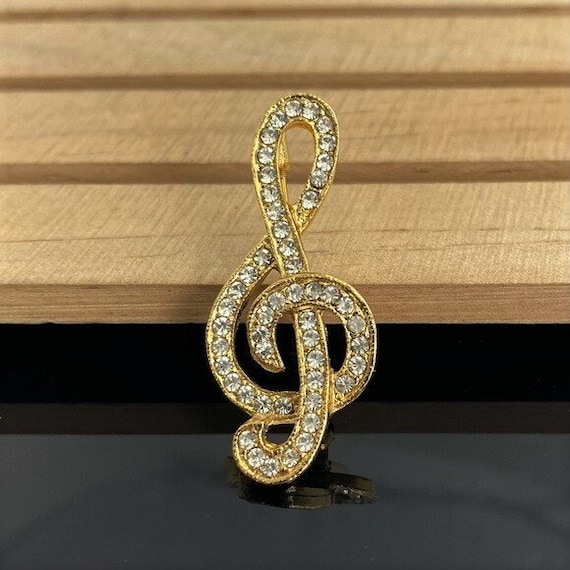This detailed photograph captures a close-up of a musical note-shaped piece of jewelry, possibly a pin, brooch, earring, or pendant. The jewelry features a gold outline, filled with numerous tiny, silver-colored diamonds that cover the entire musical note figure, giving it a luxurious and sparkling appearance. The piece is meticulously encrusted, with more than two dozen diamonds that seem to be intact and authentic. The jewelry stands centrally on a black pedestal, set against a black table. Behind it, there are three distinct brown wooden planks, providing a contrasting background that emphasizes the brilliance of the piece. The overall image showcases this exquisite piece of jewelry in sharp detail, highlighting its intricate craftsmanship and elegant design.